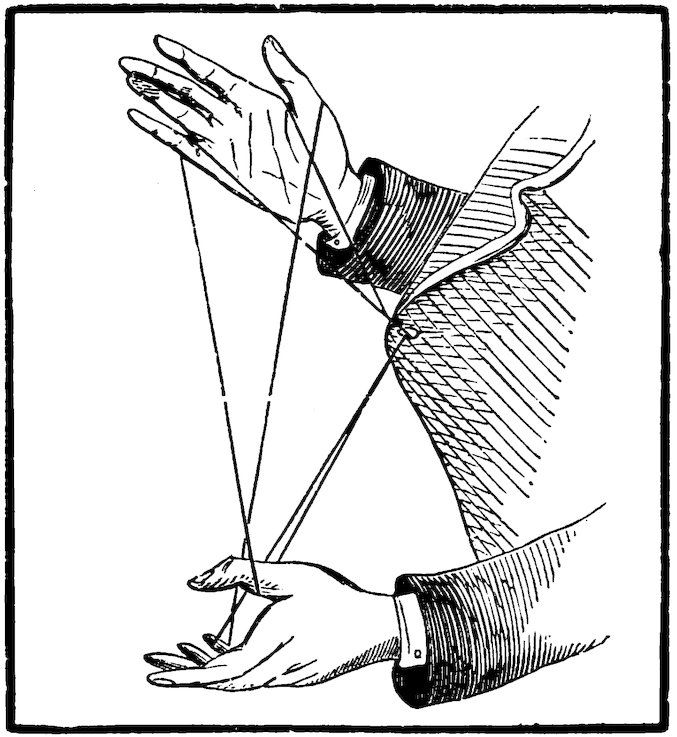This vertically aligned, black-and-white drawing features a meticulously detailed depiction of a person's hands engaged in a sewing activity. The image, framed by a solid black border, portrays a man's jacket with black cuffs and white sleeves visible beneath. The focus is on two hands positioned along a central vertical axis: the right hand is at the upper portion of the image, palm down, and the left hand is towards the bottom, palm up. Both hands are intricately involved with the string, which threads through a buttonhole on the jacket, creating a complex pattern that includes a couple of triangular shapes. The interplay of the string around the fingers and the buttonhole suggests a sewing action, emphasizing the craftsmanship involved. The drawing is executed entirely in black and white, adding a stark, classic contrast that highlights the delicate details of the hands, string, and fabric.